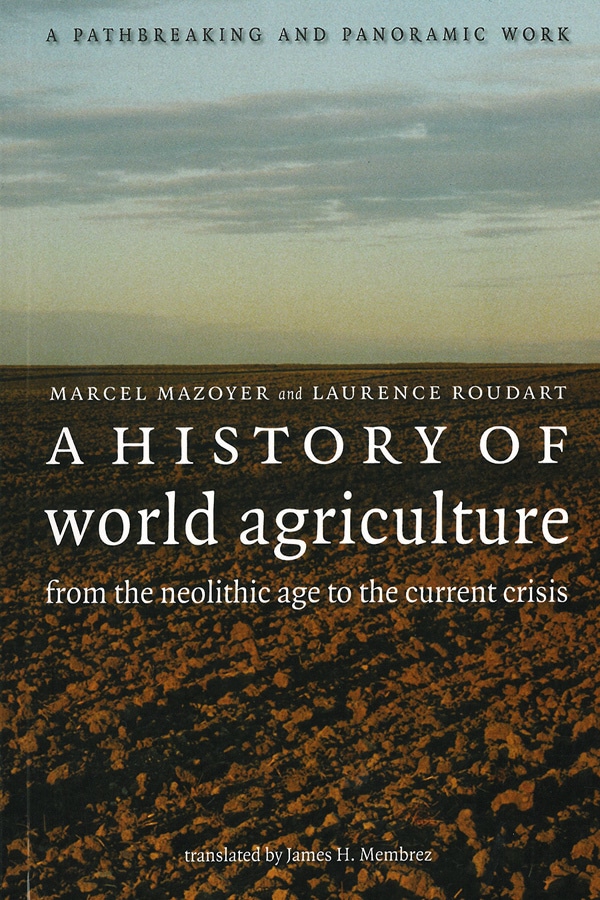This detailed book cover features an image of an agricultural field with rich, brown soil in the lower half and an orange-tinted sky with scattered clouds in the upper half. On the left side of the cover, a vertical vine runs from top to bottom. At the top of the cover, the phrase "A path-breaking and panoramic work" is prominently displayed in black text. Below this, the names of the authors, Marcel Mezoia and Lawrence Ruddart, are printed where the land meets the sky. Centered prominently in bold text is the title, "A History of World Agriculture: From the Neolithic Age to the Current Crisis." At the bottom of the cover, it notes that the book has been translated by James H. Membres. The overall design is organized and effectively captures the essence of agricultural history through a striking yet simple visual representation.